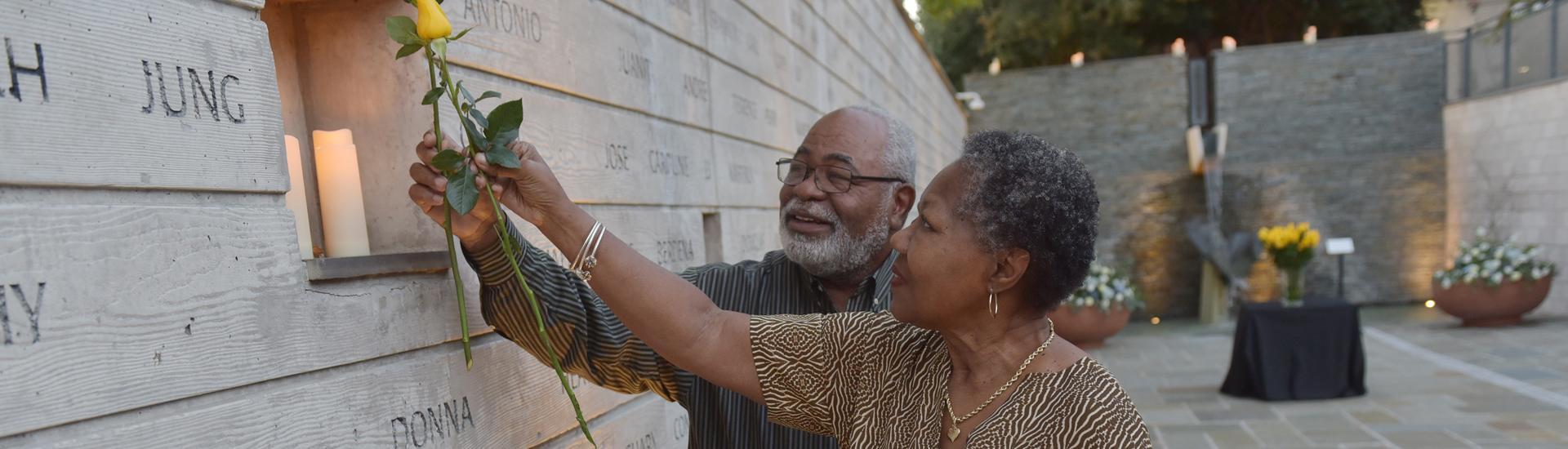This outdoor photograph, taken on a sunny day, captures a serene memorial site characterized by its expansive gray wall adorned with engraved names such as "John," "Donna," "Jose," and "Antonio." The wall features multiple small cutout windows where people have placed lit white candles. Towards the center of the image, an elderly African-American couple stands before one of these cutouts, holding yellow roses with gentle smiles on their faces. The man sports a gray beard, glasses, and a long-sleeve striped shirt, while the woman, adorned with a golden earring, necklace, and bracelet, wears a black and gold print pattern shirt. Below their outstretched arms, the shelf features the engravings "Young" and "Donna." In the background, a courtyard with tiled stone flooring unfurls, hosting a black table draped in a black tablecloth, topped with a bouquet of yellow roses. Flanking this serene setting are two large planters filled with white flowers, further enhancing the peaceful ambiance. Trees rise above the central wall, adding a natural backdrop to the solemn yet candid moment.